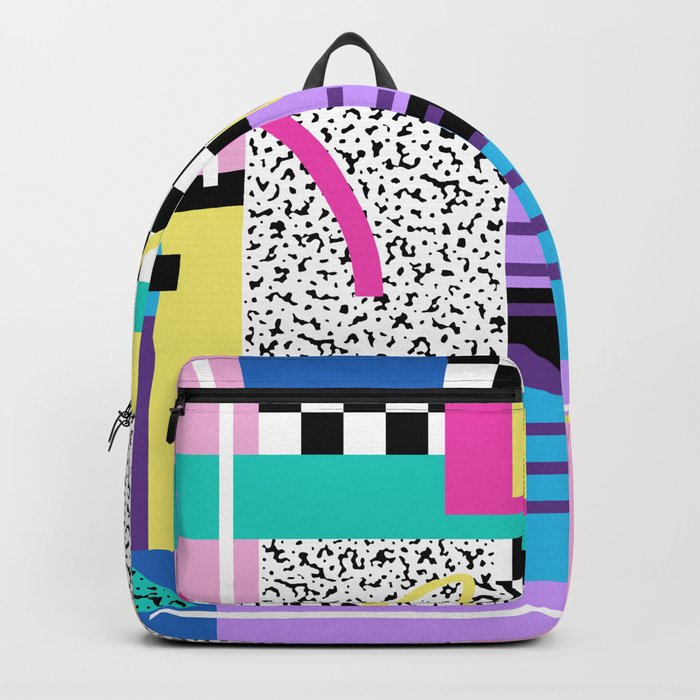The image showcases a retro, 80s-inspired backpack, positioned centrally against a subtly textured, light gray background with a slight drop shadow that adds dimension. The backpack is characterized by its curved top and rectangular bottom, suggesting a standard size likely suitable for kids, potentially appealing to girls due to its vibrant color scheme. The central section of the backpack features a distinct white stripe adorned with a black spotty design, reminiscent of the classic "marble notebook" pattern, albeit in a brighter version. Surrounding this central design, the backpack flaunts a lively array of pastel and neon colors, including teals, pinks, blues, purples, yellows, and blacks. These colors are presented in geometric shapes and lines, evoking a playful, nostalgic charm that reflects the aesthetic of the 80s and early 90s.